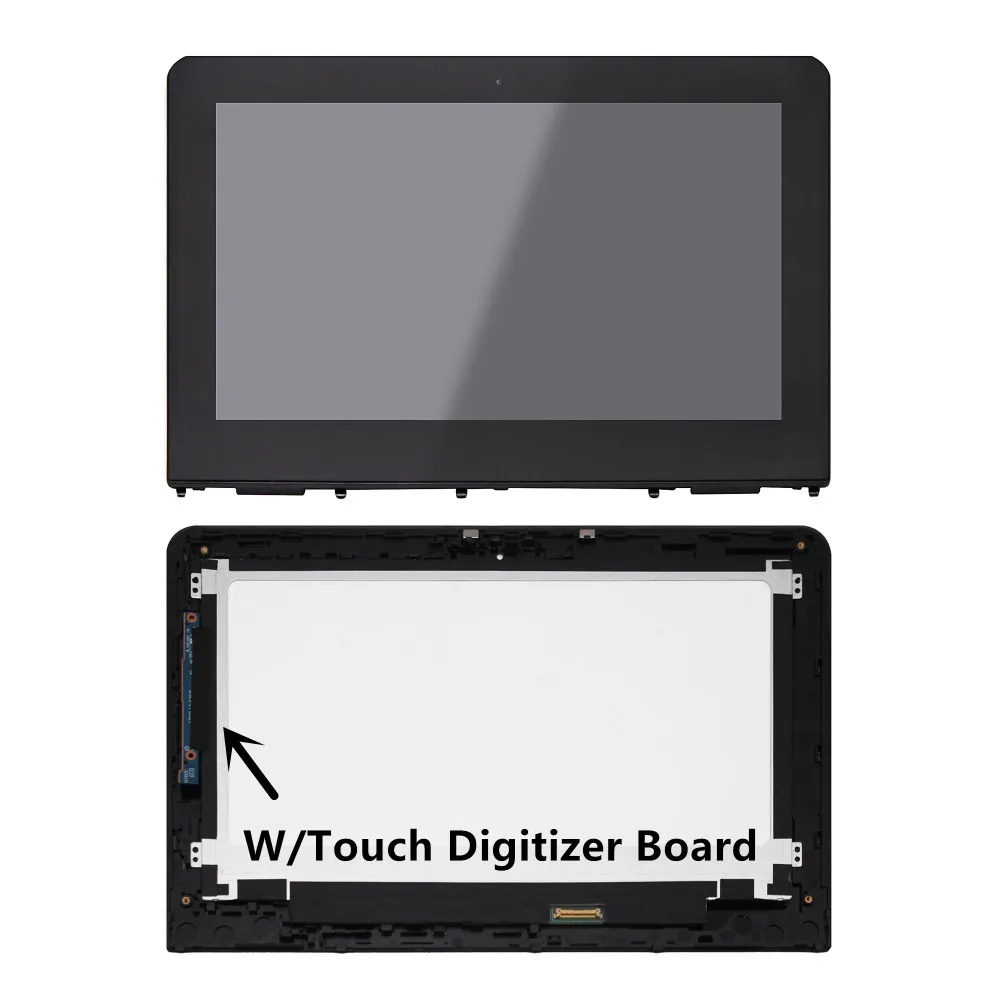This color photograph, set against a white background, provides an intricate view of a disassembled tablet. The image is split into two halves. The top half showcases the tablet's front with a blank, gray screen encased in a slightly darker gray plastic frame, featuring small clips protruding at the bottom edge where it would normally secure into place. The bottom half of the image reveals the tablet's internal components. Dominating this section is a white board with peripheral plastic edges and a circuitry area on the left, which is highlighted in blue. An arrow labeled "W/ Touch Digitizer Board" in black text points towards this blue section, suggesting it is the touch digitizer board. The image captures both the exterior and interior of the tablet, providing a detailed look at its construction and components.